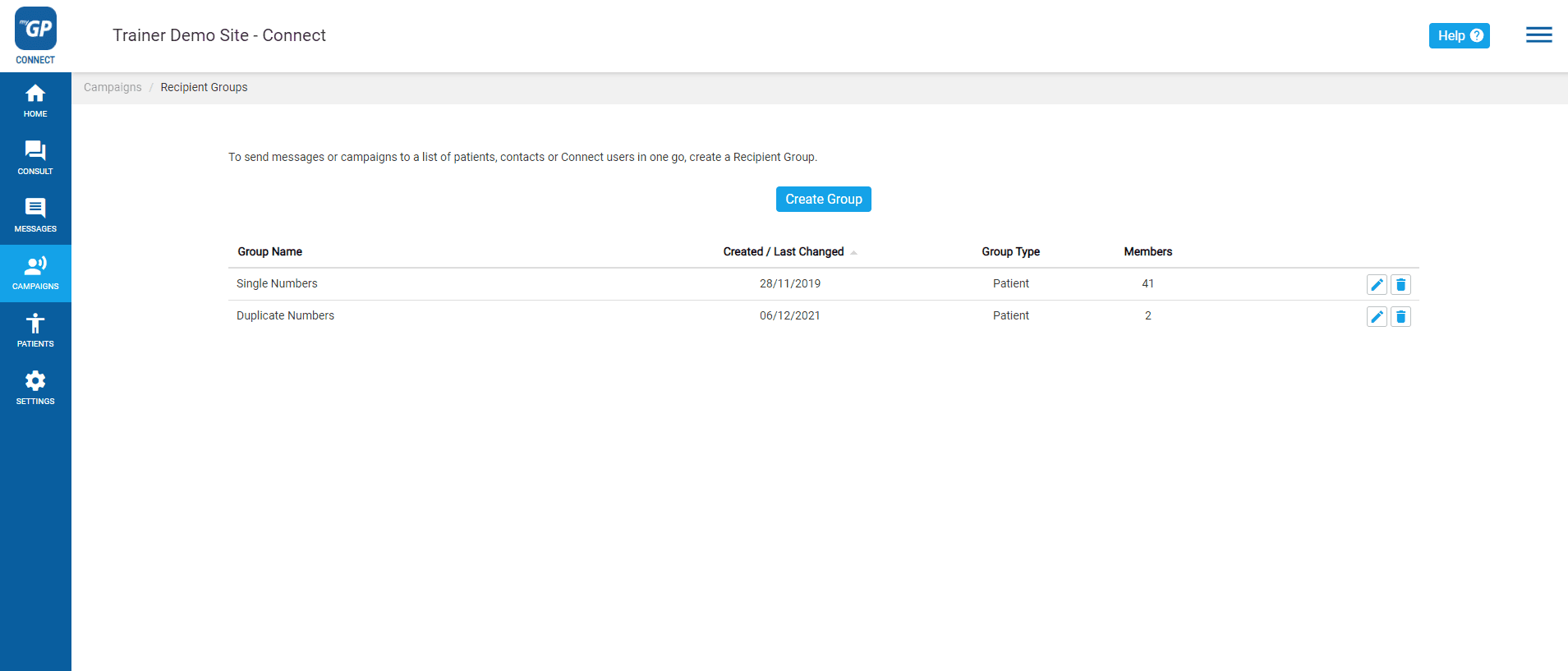A detailed screenshot appears showcasing a data table from a platform identified as "GP Connect Trainer Demo Site." The table provides structured information across several columns including "Single Numbers," "Duplicate Numbers," "Created," and "Last Change." Under the "Single Numbers" column, it indicates the creation date as "28-11-2019" and the last change being "Past the Single Numbers." The "Group Type" is listed as "Patient Members 41." Meanwhile, under the "Duplicate Numbers" column, the creation date is "6-12-2021" with a "Group Type" indicating "Patient Members 2." The context suggests this might be a demo site used for training purposes, possibly in the medical or healthcare domain, given the references to patient groups and numerical records.